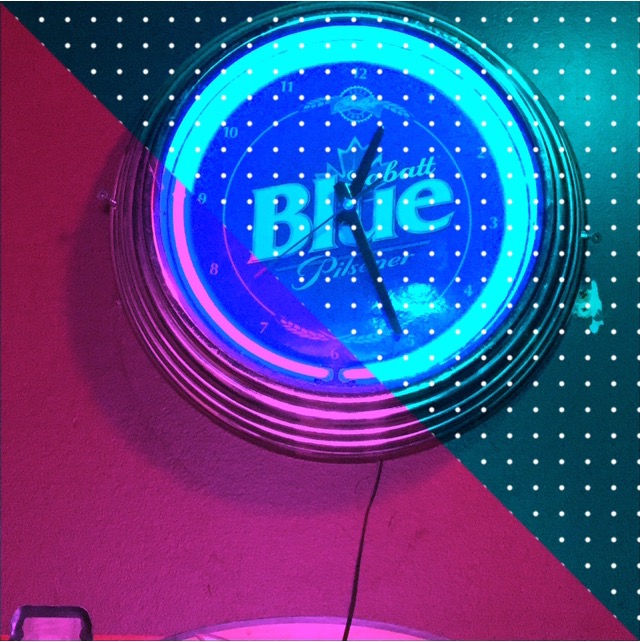The photograph captures an indoor scene centered on a wall-mounted clock. The wall is uniquely decorated, divided diagonally into two contrasting colors: a bright pink on one side and a dark blue with white dots on the other. This striking split runs directly from the upper left to the lower right of the image, creating a dynamic and visually engaging backdrop.

The clock, the focal point of the image, features a sleek silver reflective border and a vibrant blue face adorned with the words "Blue Pilsner" in white lettering at its center. The clock's hour markers are also denoted in white numbers, while the minute, hour, and second hands are black, offering a sharp contrast to the vivid blue background.

Emerging from the bottom of the clock is a black cord, suggesting it is an electric model rather than battery-operated. The lower portion of the image reveals the edges of several indistinct objects in silver, white, and black hues. Due to the limited view, these items remain unidentified, adding an element of intrigue to the composition.

This detailed description captures the essence of the photograph, highlighting the unique color scheme, the clock's design features, and the subtle mystery of the partially visible objects.